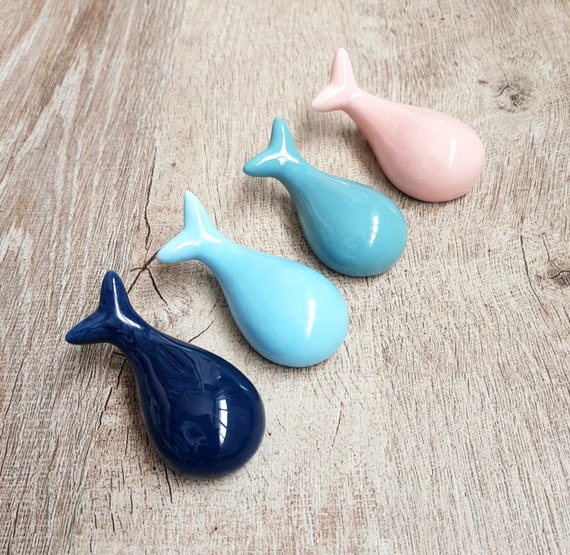This image captures a set of four ceramic chopstick holders, each shaped like simplified fish or small whales, arranged diagonally on a light brown wooden surface with hints of white. From the bottom left to the top right, the ceramic figures are positioned with their circular heads angled downward to the right and their tails pointed upward to the left. The first holder is a dark, almost black, blue with a shiny finish. Next is a lighter robin's egg blue, followed by a vivid teal reminiscent of tropical ocean waters. The final holder is a delicate light pink similar to rose quartz. Each piece has a sleek, teardrop design without any facial features, emphasizing their elegant and minimalist form.